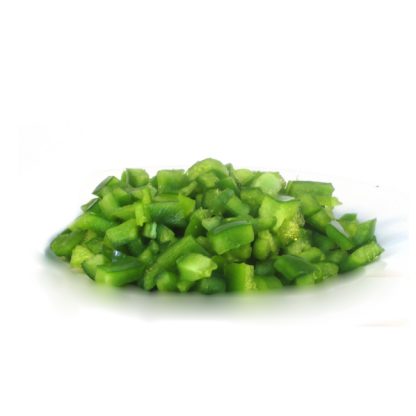This color photograph, in landscape orientation, presents an image of bright green bell peppers that have been meticulously diced into small, bite-sized chunks and piled into an oval-shaped mound. The pile likely consists of pieces from two or three peppers, with their dark green exterior transitioning to a lighter green interior where the flesh is. The peppers have been carefully prepared with no seeds or stems visible, emphasizing the rich green hues. The background display is pure white, devoid of any context such as a plate or cutting board, giving the impression the pile is floating. A slight gray drop shadow beneath the pile enhances this floating effect, contributing to a minimalist but highly detailed focus on the vibrant peppers. The photograph employs a realistic, representational style common in food photography, perhaps with some filters applied to accentuate the striking greens of the vegetable.